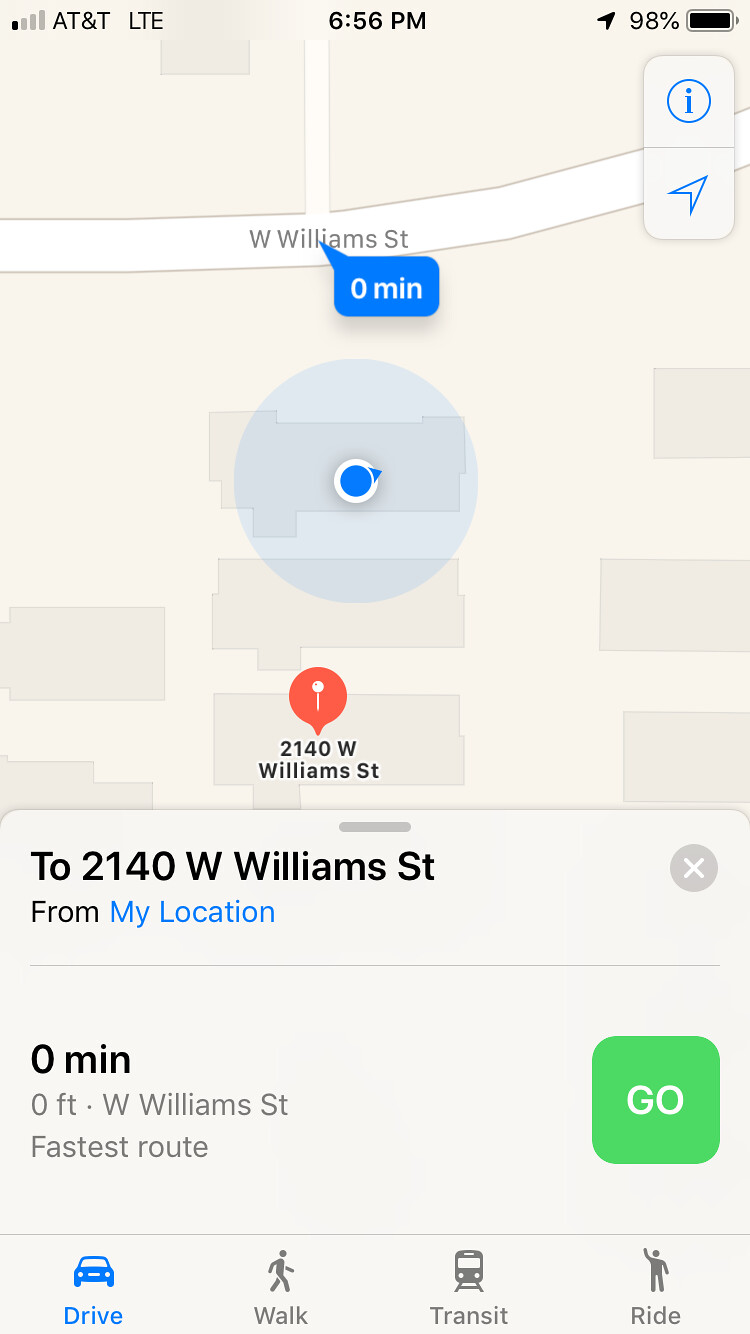This image is a screenshot from a MAPS program on a cell phone. At the top of the screen, the status bar displays "AT&T LTE," the time is "6:56 PM," and the battery is at "98%."

The map prominently shows a specific location on West Williams Street. A red pin marks "2140 W. Williams Street" with an arrow pointing to the exact spot. Above the street name "West Williams Street," there is a blue rectangle with rounded corners, indicating "0 minutes."

At the bottom of the screen, detailed navigation options are presented. It reads "0 feet West Williams Street fastest route," and next to this information is a green square with rounded corners and the word "GO" in white text.

Moreover, the bottom navigation bar offers different travel options: "Drive" has a blue car icon, "Walk" is represented by a walking person, "Transit" with a bus icon, and "Ride" with a person waving their hand.